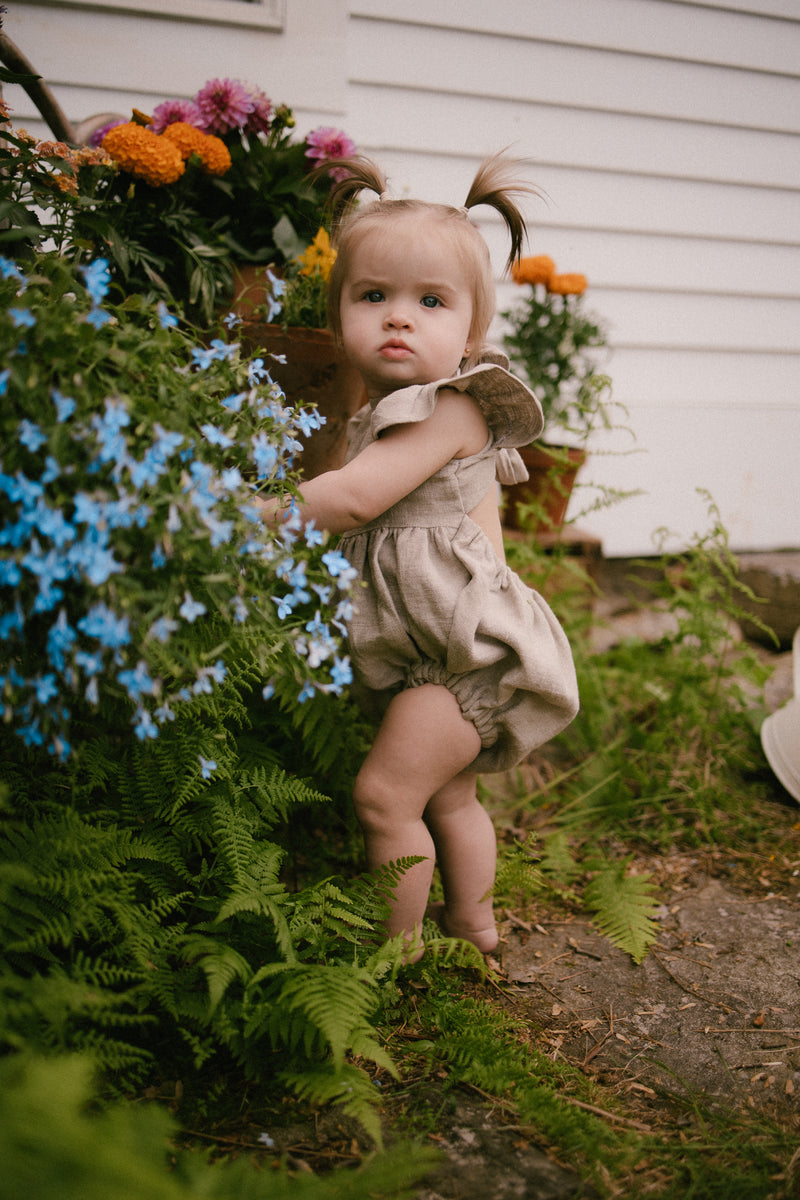The photograph captures a mischievous-looking toddler girl standing in a vibrant garden in front of a house with white or tan siding. The focal point of the image is the little girl, who is facing left but looking toward the camera with a curious and playful expression. She is dressed in a beige ruffled romper and has her hair styled in two pigtails. Her chubby legs are bare, and her left leg is bent as she reaches into a bed of flowers, her hands obscured. The garden around her is lush with various flowers, including eye-catching little blue flowers arching over her head, alongside orange, purple, yellow, and pink blossoms. The ground beneath her is a mix of dirt and green grass. The composition of the photograph beautifully contrasts her innocent yet mischievous demeanor with the colorful, lively flora surrounding her.